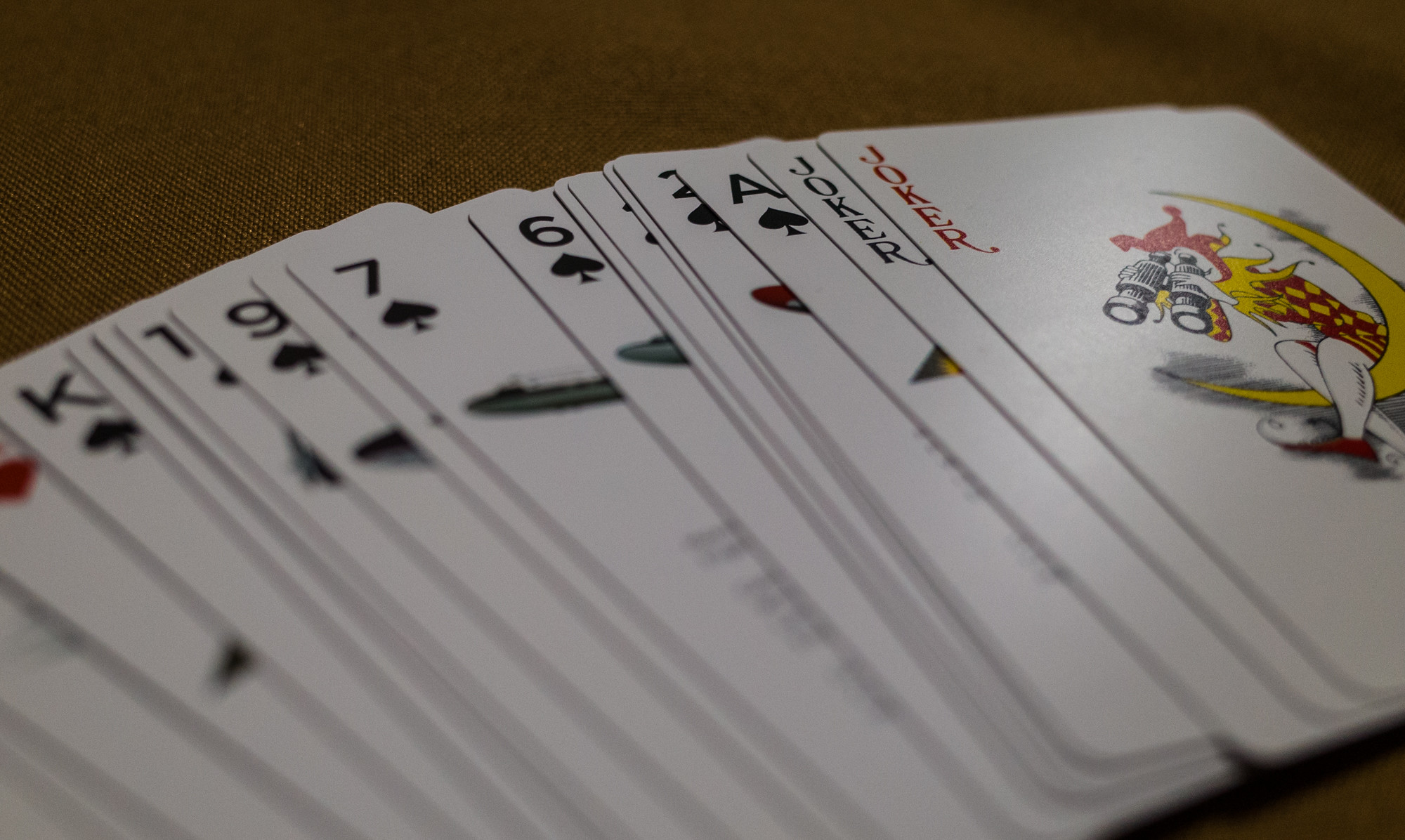In this photograph, a selection of playing cards is scattered across a table in a seemingly random arrangement. Among the cards, several belong to the spade suit, including a few that hint at a possible sequence. Two joker cards are prominently displayed within the spread. Of note is the red joker card, which is the only card fully visible, positioned at the far right of the array. This card features a whimsical jester character perched on a crescent moon, peering through binoculars. The jester is adorned in a vibrant red cap and a red and yellow outfit, complete with a decorative yellow fringe around the neck.